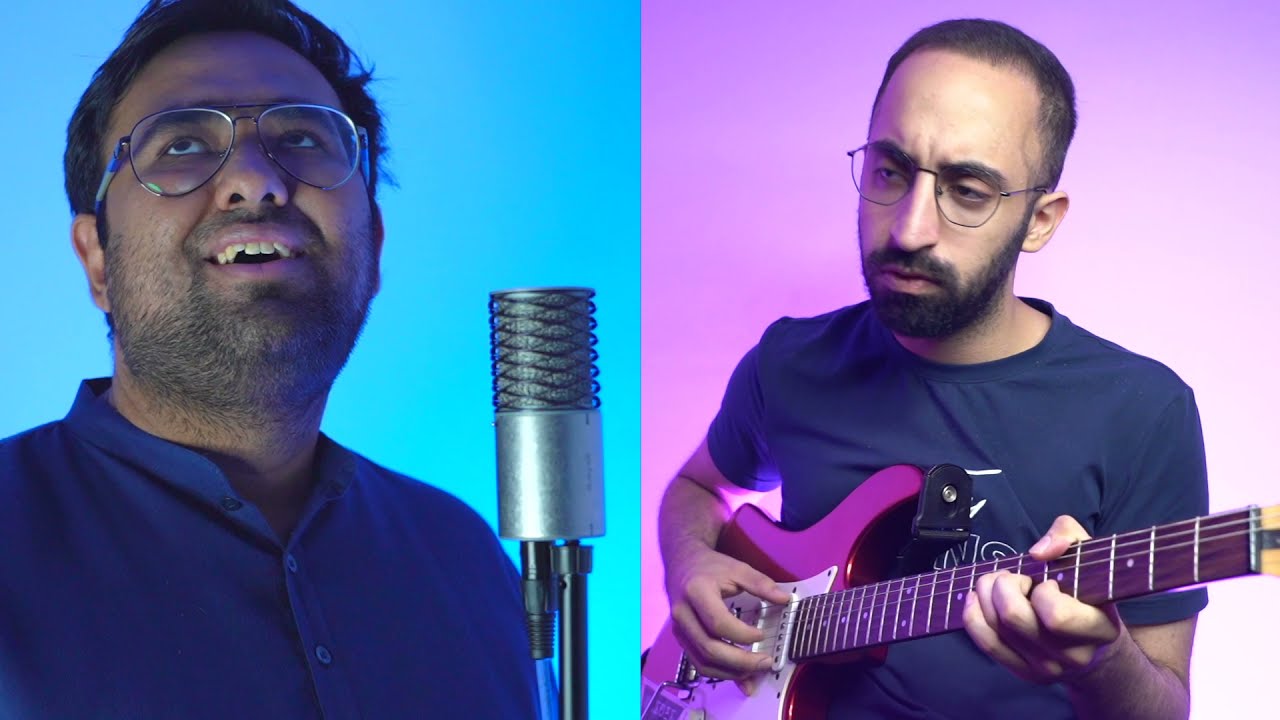The image is split into two sections. On the left, there is a man with light brown hair, combed to his left, wearing silver-framed glasses that are slightly square yet circular, reminiscent of 70s style. He has a scruffy beard covering his chin and cheeks, and he's dressed in a blue long-sleeve shirt with only the top button unbuttoned, revealing a circular neckline. The background behind him is a light sky blue. He appears to be looking upwards, smiling slightly, with a microphone positioned to his left, indicating he might be singing.

On the right side, there is a more serious-looking man with short brown hair, styled to his right. He sports a black, well-groomed beard and wire-frame circular glasses. He is wearing a blue short-sleeve t-shirt and is strumming a pinkish-purple electric guitar with his right hand. The background behind him is a light purple that complements the color of the guitar, suggesting a consistent lighting or thematic choice.

Together, the two men seem to form a cohesive scene, likely collaborating in a musical performance or production.